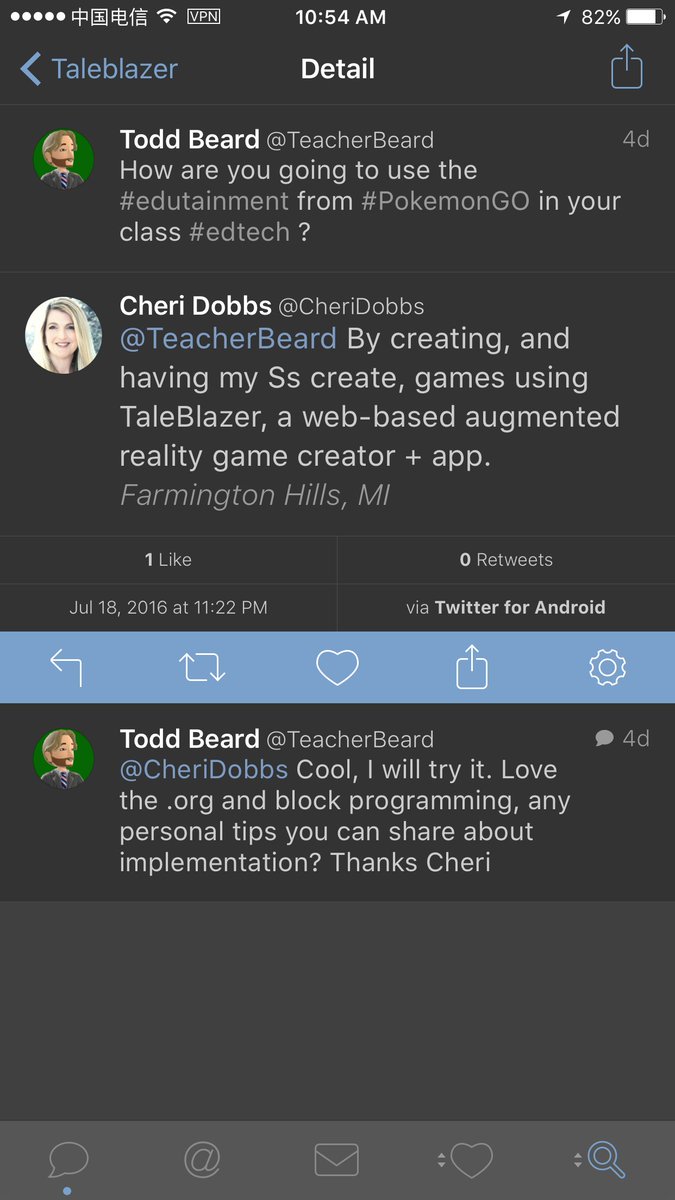**Caption:**

The image shows a tweet from a user discussing the integration of Pokemon Go and educational technology in a classroom setting. The UI elements visible include three bars for Wi-Fi signal strength and Asian script indicating VPN usage. The status bar displays the time as 10:54 AM, with a GPS indicator and a battery level at 82%. Below this, the screen shows an interface with various icons and text, including a blue arrow pointing left labeled "tailblazer," and a blue square labeled "upload."

The tweet features a user, identified by their handle "Todd Beard," discussing the creation of games using "Trailblazer," a web-based augmented reality (AR) game platform. The tweet mentions specific hashtags like #EdTech, #GoPokemonGo, and #entertainment. 

The shared content originates from Farmington Hills, Michigan, with the user providing insights about incorporating AR into educational programs for students. The tweet is accompanied by interaction icons: an envelope (for direct messages), a heart (for likes), and a magnifying glass (for search), all set against a variegated background.